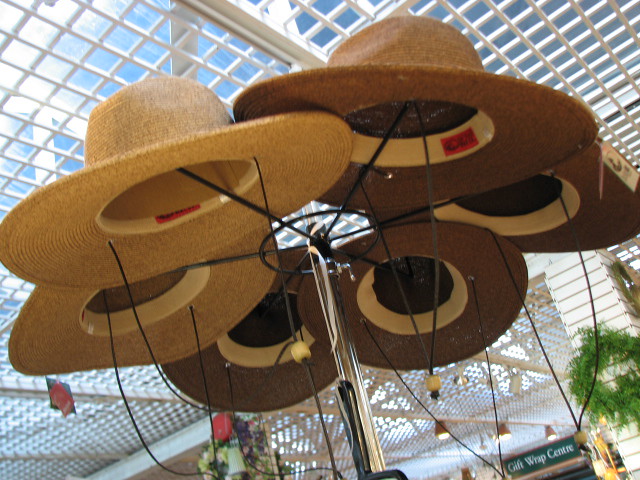The image depicts a black wired hat rack holding six hats, likely sombreros or straw sun hats, with a rough wicker texture. The hats come in shades of light tan and dark brown, each equipped with black strings and adjustable beads for securing under the chin. The scene appears to be in a shopping setting, possibly a mall, flea market, or nursery, and is captured from a low angle. Above, a white, cage-like, grated ceiling is visible, and in the background, there are green tree branches and various decorative wreaths. On the distant right side, a sign reading "Gift Wrap Centre," spelled in British English, suggests a possible UK or European location.